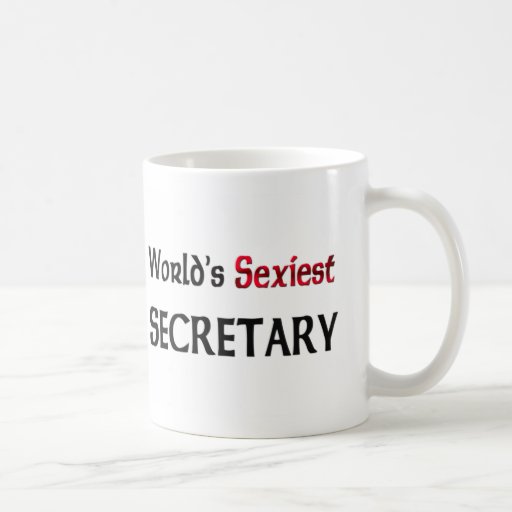The image features a standard-sized, glossy white ceramic coffee mug prominently displayed on a white and gray marble tabletop. The handle of the mug, which is proportionally large and extends close to the top and bottom of the cup, is also white. The background behind the mug is a plain white wall, which, combined with the white mug and marble surface, results in a highly washed-out aesthetic dominated by the color white.

The mug bears a bold and somewhat controversial message: "World's Sexiest Secretary." This text is arranged in three lines, each with distinct typography. The word "World's" appears at the top in black, with an initial capital 'W' followed by lowercase letters and an apostrophe. The middle word, "Sexiest," stands out with a primarily red color that includes a subtle gray-black gradient in the center; it is written with a capital 'S' followed by lowercase letters. The final word, "SECRETARY," is situated at the bottom in all uppercase black letters. The text decorates the side of the mug, lending it a somewhat provocative flair.